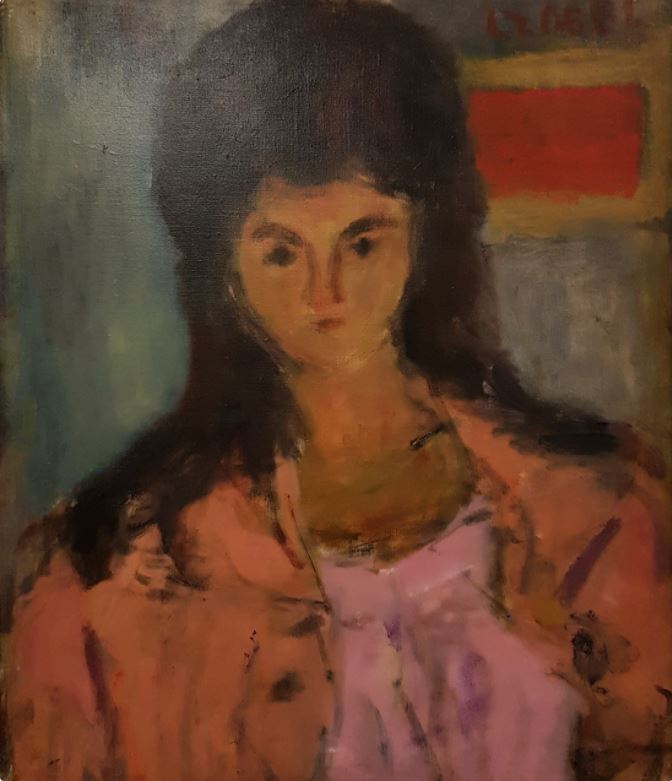This painting depicts a woman with voluminous, wild brown hair, styled shorter around her face and longer in the back, reminiscent of an 80s American look. Her head is tilted downward, causing her chin to tuck close to her neck. She has dark eyes, prominent brown eyebrows, and a very small, pursed mouth. Her attire includes a peach-colored blazer layered over an open v-neck top, which transitions in color from pink to white with purple and pink hues suggesting a spill or gradient effect. The background is a washed-out bluish-gray, and to the right of her head, there is a red rectangle with a yellow border. The painting, with its lack of hard lines and detailed features, evokes a hazy, almost dreamlike quality, emphasizing the woman's broad shoulders and the ambiguous detailing of her earrings and jacket pockets.